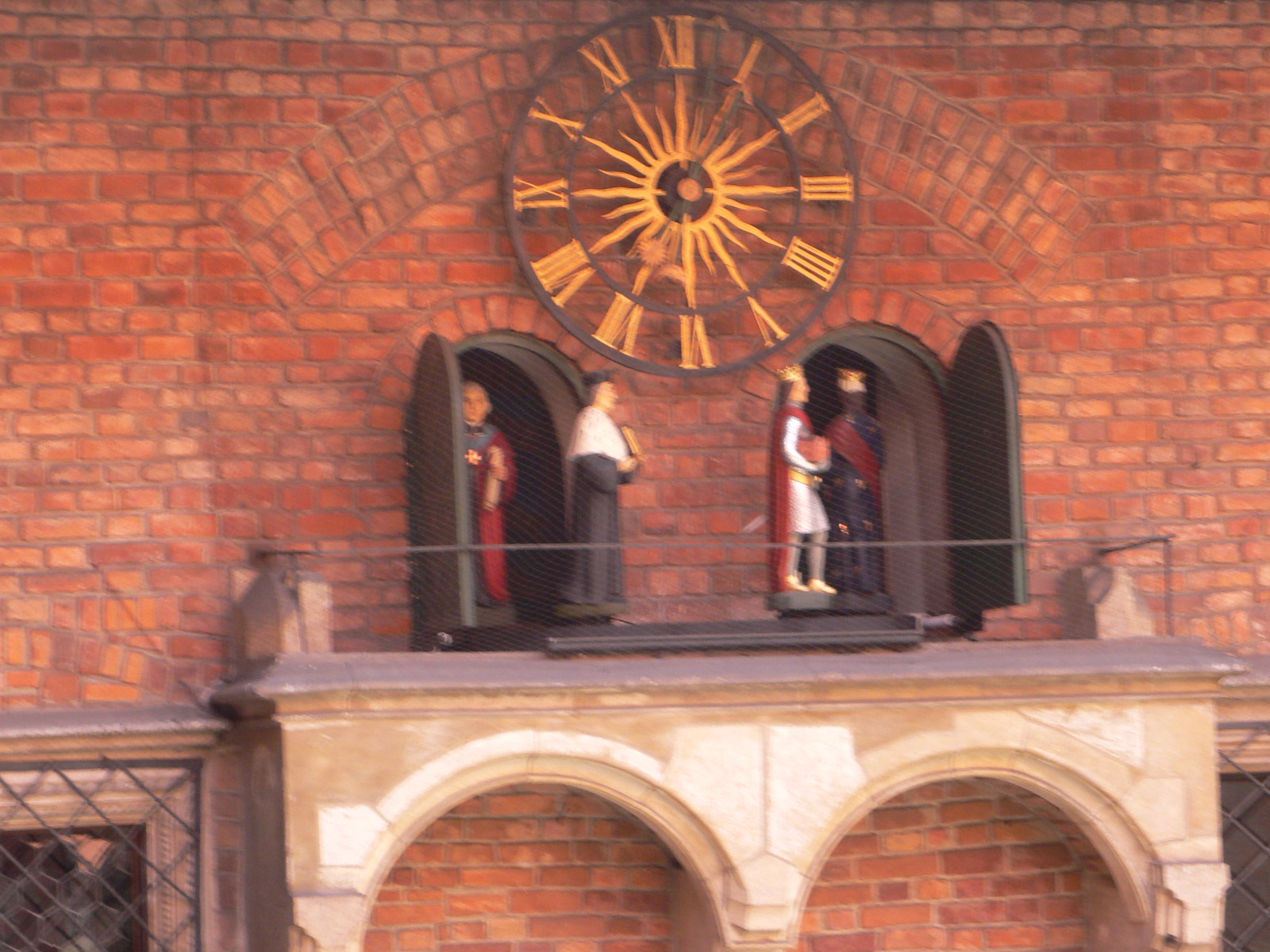This photo captures a large, ornate clock mounted on the brick exterior of a building, likely a church or a significant town square structure. The clock is designed with intricate black metal cutouts, highlighted with gold Roman numerals, and features a radiant sun motif at its center. Below the clock face are two arched doors, flanked by partial stone archways and protective metal screens. These doors open to reveal a rotating mechanism presenting religious figures in robes and crowns, who emerge from one door on pedestals and walk into the other. Despite the blurry quality of the image, details such as ceramic edges of nearby windows and the brick detailing behind the clock are visible, enhancing the historic and architectural charm of the scene.